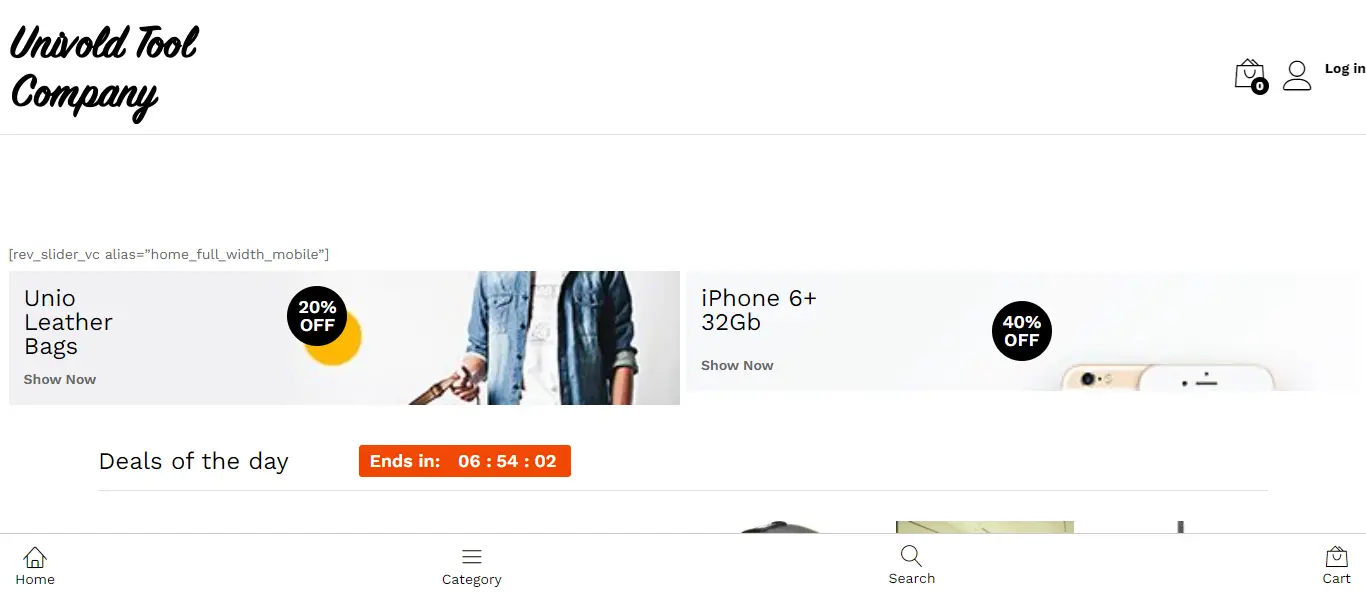In the screenshot set against a solid white background, the upper left corner features "Ununivold Tool Company" in elegant black cursive block lettering. Directly beneath this is an image capturing a man's chest without showing his head or legs. The man is dressed in a white shirt layered with a button-down denim long sleeve shirt, which has the sleeves rolled up. He holds a leather strap in his right hand. To the left of this image, text reads "20% off Unio Leather Bags, shop now," with a smaller text above in parentheses stating "Rev Slider VC Elias = Home Full Width Mobile." In the upper right corner, a shopping bag icon shows zero items with a login option beside it. To the right of the man’s shirt, "iPhone 6 Plus 32 GB, shop now" is prominently displayed. Beneath this, there is a countdown for a promotional offer stating "Deals of the day ends in 6 hours 54 minutes 2 seconds."